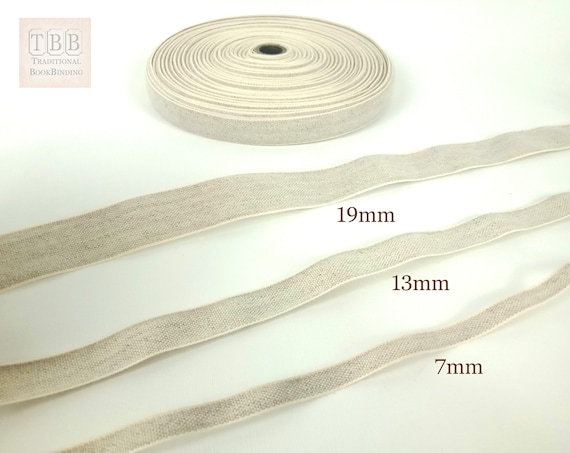This landscape-oriented color photograph showcases traditional book binding materials arranged in a meticulously organized composition. At the top left corner, set against a beige background, is an octagonal logo bearing the letters "TBB," under which the phrase "traditional book binding" is inscribed. Centrally positioned at the top, a coil of book binding tape, primarily white in color, lies flat, providing a focal point with a slight overhead viewing angle. Below this coil, three unrolled strips of book binding tape extend diagonally from the left to the right of the image. Each strip is distinctly annotated with black text specifying its width: 19mm at the top center, 13mm beneath it but slightly more to the right, and 7mm at the bottom right. The photograph, rendered in a style that combines realism with text, aims to visually educate on the varying widths of the book binding materials. The entire scene is set against a white and grey background, enhancing the clarity and contrast of the components, making it an exemplary piece of product photography.